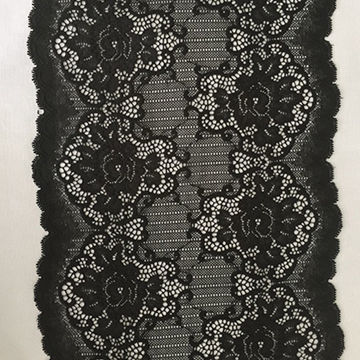The image showcases a detailed view of a piece of intricate, black lace fabric set against a light gray background. The fabric, occupying the majority of the rectangular frame, features ornamental, ruffled black edges. Centrally positioned, the lace fabric is adorned with two vertical columns of black squiggly lines that interconnect. These lines are bordered by an ornate pattern of white and black, resembling floral shapes with black curved lines stemming from the borders. The floral-like shapes, appearing as three units in each column on both sides, are set against a speckled gray and white background. The overall composition creates a visually captivating pattern with a combination of ruffled edges and an elaborate lace design.